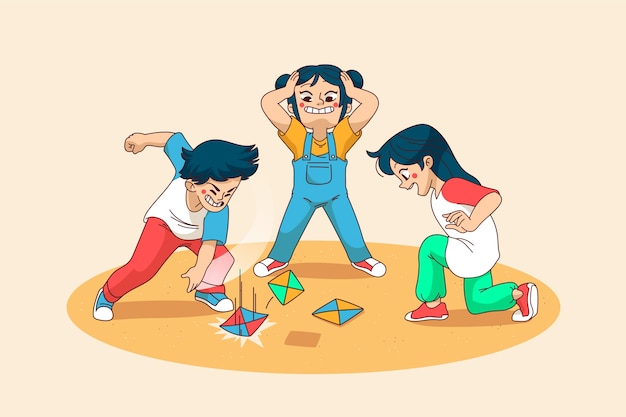In this vividly detailed cartoon illustration with an anime art style, three children are depicted engaging in a lively game on an elliptical area of light orange-brown, almost peach-colored, that contrasts with the cream-colored background. The scene captures their dynamic poses and expressions as they play a paper snap game. 

On the left, a young boy is crouched forward, fervently slamming a square paper piece with red and blue diamond patterns onto the ground, displaying a triumphant grin. He is dressed in a white t-shirt with blue sleeves and red pants. His intense action is surrounded by black lines, emphasizing the snapping impact.

To his right, the central figure, a girl with black pigtails, stands in shock, her hands dramatically clutching her head. She wears a gold t-shirt beneath blue overalls and red sneakers, her wide eyes and open mouth accentuating her astonishment.

On the far right, another girl, happy and seemingly approving of the boy’s successful slam, kneels on one knee. She has long dark hair and is attired in a white jersey with red sleeves, bright green shorts, and red sneakers. Her hand rests on the floor, and she observes the outcome with a satisfied expression. 

Beside them lie two other paper squares, unturned and indicative of previous unsuccessful attempts. The entire scene is brought to life through vibrant colors and animated expressions, capturing a moment of playful triumph and camaraderie.